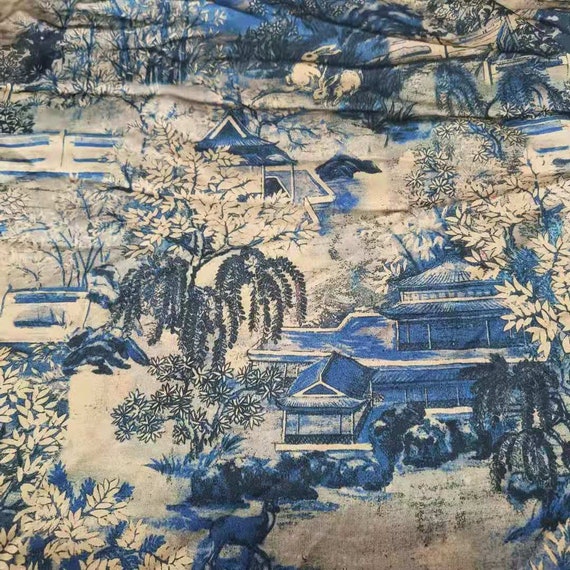The image is a detailed and serene scene, likely an old Japanese or Chinese painting, presented on what appears to be a piece of fabric, possibly a duvet cover or blanket. Set against a white background, the scene is rendered predominantly in shades of blue, from light blue to almost black. The main focus is a grand, multi-story Asian building constructed with wooden and bamboo materials and crowned with intricately curved, pointed roofs suggestive of traditional Oriental architecture. Surrounding this structure is lush vegetation, including trees with white leaves, flowering branches, and vines that contribute to a wintery, snow-kissed atmosphere. Other buildings, similarly designed with curved roofs, populate the scene, creating a sense of a serene village. The landscape is dotted with various fauna, including a painted deer crossing through the foreground and a large rabbit descending a hill in the background. The presence of streams, fences, and numerous trees with navy branches adds further depth and complexity to this tranquil, wintry scene.